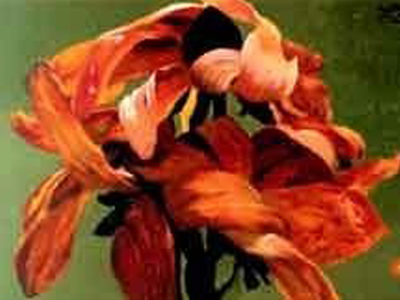The image depicts a somewhat blurry, low-resolution painting of a vibrant flower. The focal point is a close-up of the flower's blooming head, showcasing petals that vary in color from orangish-pink to darker orange, with a few hanging down and others interlocking in a circular pattern. The background features a gradient of green hues, transitioning from a lighter green-yellow on the left to a darker green on the top right. The black stem or trunk of the flower is visible, as well as a central black pod-like structure at the top. The painting includes no identifiable markers such as an artist's signature or title.